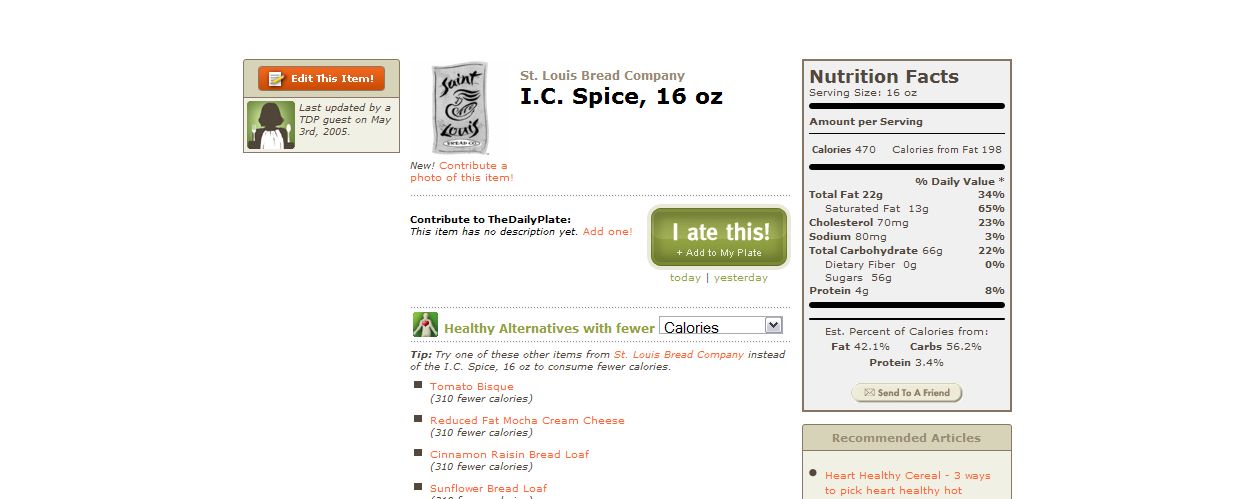This image captures an entry from an old-fashioned nutrition feedback website, featuring a nutrition label and a detailed descriptor for a product from St. Louis Bread Company named "I See Spice." The image shows a 16-ounce serving containing 470 calories and 22 grams of fat. In addition to the nutritional information, the entry is marked with an update by a guest, dated May 3rd, 2005. The website appears to provide insights on food items and suggests alternative, healthier options with fewer calories and lower fat content.